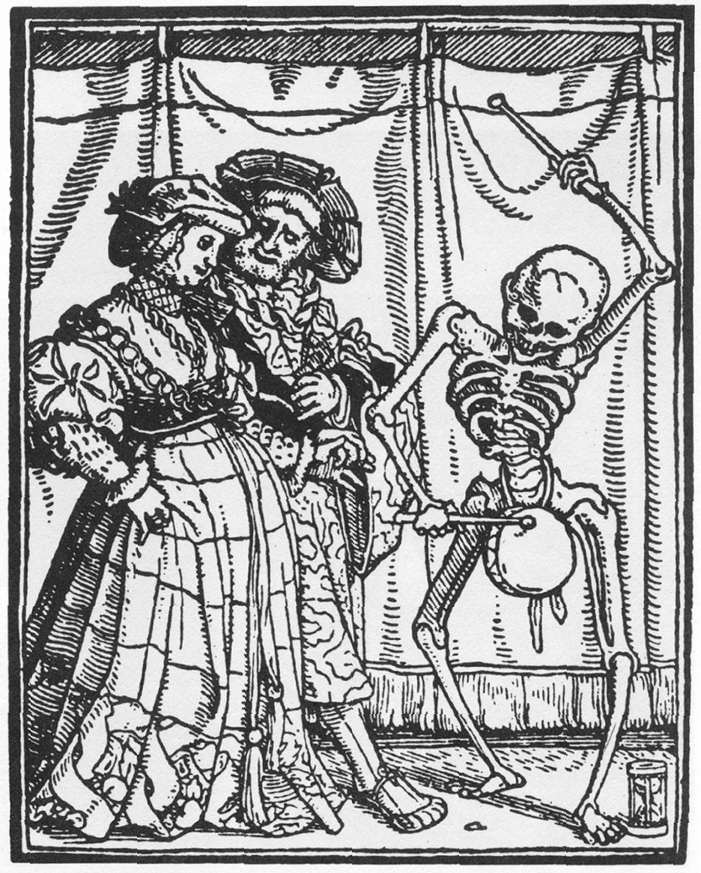This black and white rectangular pencil drawing captures an evocative scene set in an unspecified era, reminiscent of the 1700s in Europe. On the right-hand side of the image, a human skeleton is depicted dynamically playing a small round drum tied around its hips, with drumsticks in both its bony hands—its right hand striking the drum while the left is raised in the air. Below its left foot, an hourglass suggests the passage of time. Beside the skeleton, to the left, stand a middle-aged man and woman in elegant, period-specific attire. The woman, whose gaze is fixed on the drumming skeleton, wears a floor-length gown with puffy sleeves, a high neckline, a hat, a choker, and a long necklace. Her pulled-back hair and composed demeanor add to the intricacy of her depiction. Close to her, perhaps with his right arm around her, the man observes her intently, dressed in a knee-length elaborate costume with thick, hanging sleeves, an ornate cravat, and shoes with rolled-up toes. He sports a large hat, a beard, and a mustache, augmenting the historical ambience. The couple stands closely, possibly in front of a curtain or a tent, adding a mysterious backdrop to the scene.